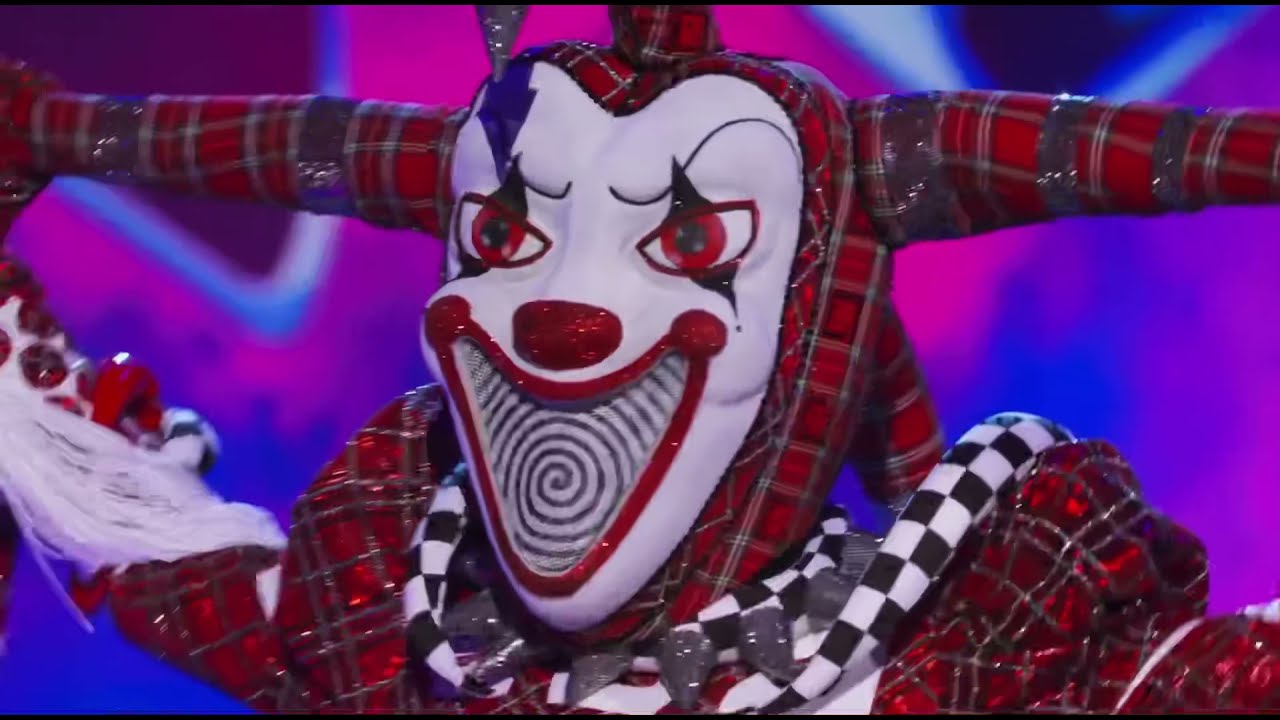The image depicts a character dressed as a sinister clown, likely from the television show "The Masked Singer." The clown's costume is elaborate and unsettling, featuring a predominantly white face with exaggerated red eyes and a glittering red nose. The mouth is styled into a hypnotic black and white spiral pattern with a striking V shape, reminiscent of the Twilight Zone. The costume is adorned with a mix of red plaid and black-and-white checkered patterns, including a checkered scarf around the neck and a stiff red plaid jacket that matches the pattern on the horns protruding from the sides of the head. Additionally, there are flannel-like designs on the face and large, puffy sleeves. The background is vibrant, with wavy purple, blue, and pink lighting, consistent with the theatrical stage setup of "The Masked Singer," where celebrities perform in disguise. The overall effect is eerie, enhanced by the clown's menacing black pupils and dark makeup accents, capturing the creepy aesthetic of a jester or a Joker-like figure.